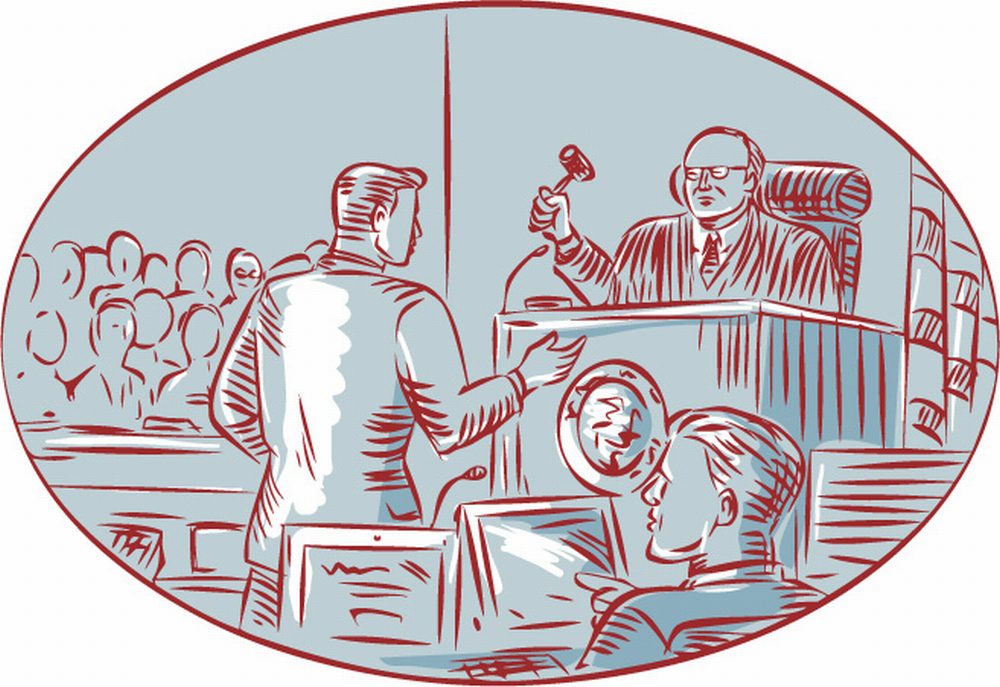This detailed caption synthesizes the shared elements across the three descriptions to provide a cohesive and thorough picture of the image:

In this detailed drawing set against a white background, the scene is enclosed within a wider-than-tall oval frame with a mauve border. The inner part of the oval features a courtroom scene sketched in a burgundy color palette, laying over a background that shades from medium to dark blue, with hints of light blue as well. At the heart of the depiction, a judge, a man with glasses, dressed in traditional judicial robes over a white shirt and tie, is poised with a gavel raised, ready to strike. Directly in front of the judge stands a man assumed to be a lawyer, who has one arm raised as if making a point; his back and side are visible to the viewer. On the right side of the foreground, another man sits behind an array of what appear to be computer monitors. To the left of the lawyer, possibly a jury or observers, their forms are sketched out in minimal detail, visible only from the shoulders up. The vivid burgundy lines against the blue background add a stark contrast, highlighting the activity and tension of the courtroom scene.